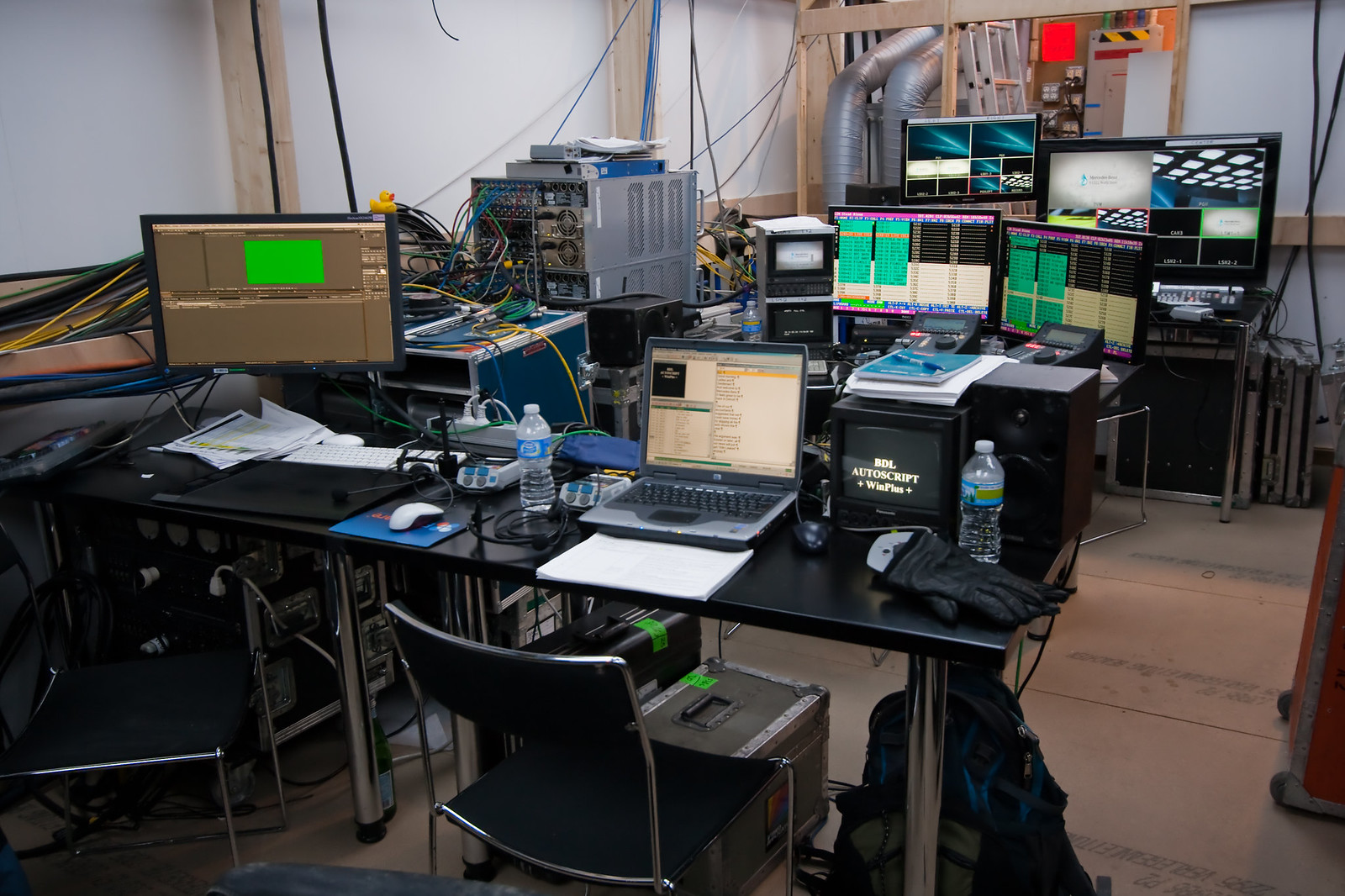The photograph depicts a makeshift IT workshop, possibly for a startup business or an IT department set up in a hurry. The room appears to be unfinished, and the setting might be a construction area, storage area, attic, or basement. The floor looks like concrete backer board or cardboard, and the walls are exposed studs, with visible ductwork for heating and air conditioning.

There are several tables cluttered with electronic equipment, including at least five or six flat-screen computer monitors, laptops, and various measuring instruments and readout machines. The presence of numerous cables strung across the room adds to the chaotic appearance. Underneath the tables, there are equipment boxes, potentially containing tools or other necessary devices.

Despite the seemingly hasty setup, the room serves as a functional workspace with multiple workstations outfitted with chairs and water bottles, indicating active use. Large server towers and other significant electronic apparatus dominate the background, reinforcing the impression of a dedicated but ad hoc command center focused on IT tasks or computer technology operations.